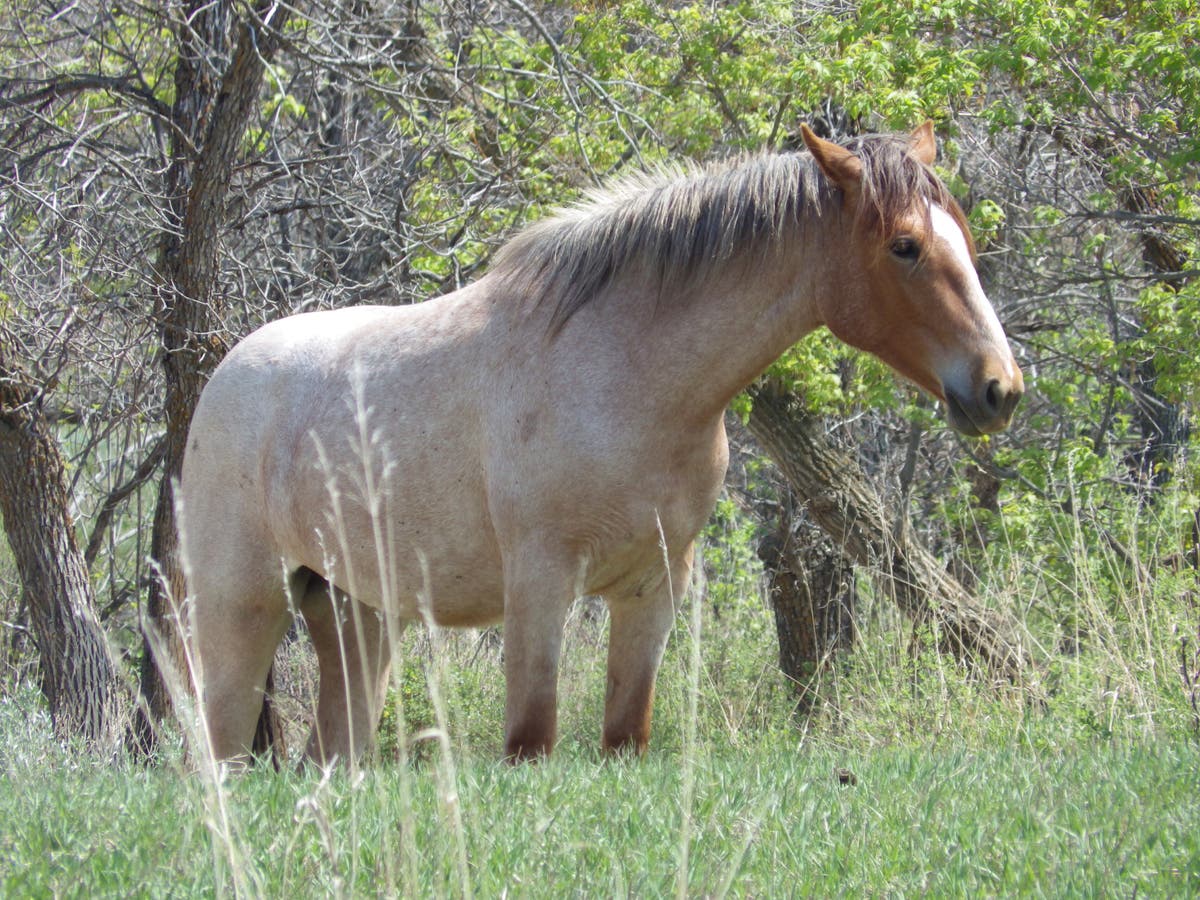In this picture, we see a beautiful horse standing knee-deep in a grassy field, surrounded by a grove of trees that still have a hint of green in their leaves. The horse has a light brown and white coat, notably not spotty, with a mane that is almost grayish-white or gray-brown. Its face is a distinct reddish-brown, darker than its body, and features a white stripe running from the middle of its forehead down to its nose. The horse, standing still with its head slightly raised, appears content and possibly focused on digesting the grass it has been munching on. The scene is peaceful, with the tranquil horse blending harmoniously into its semi-forest surroundings.